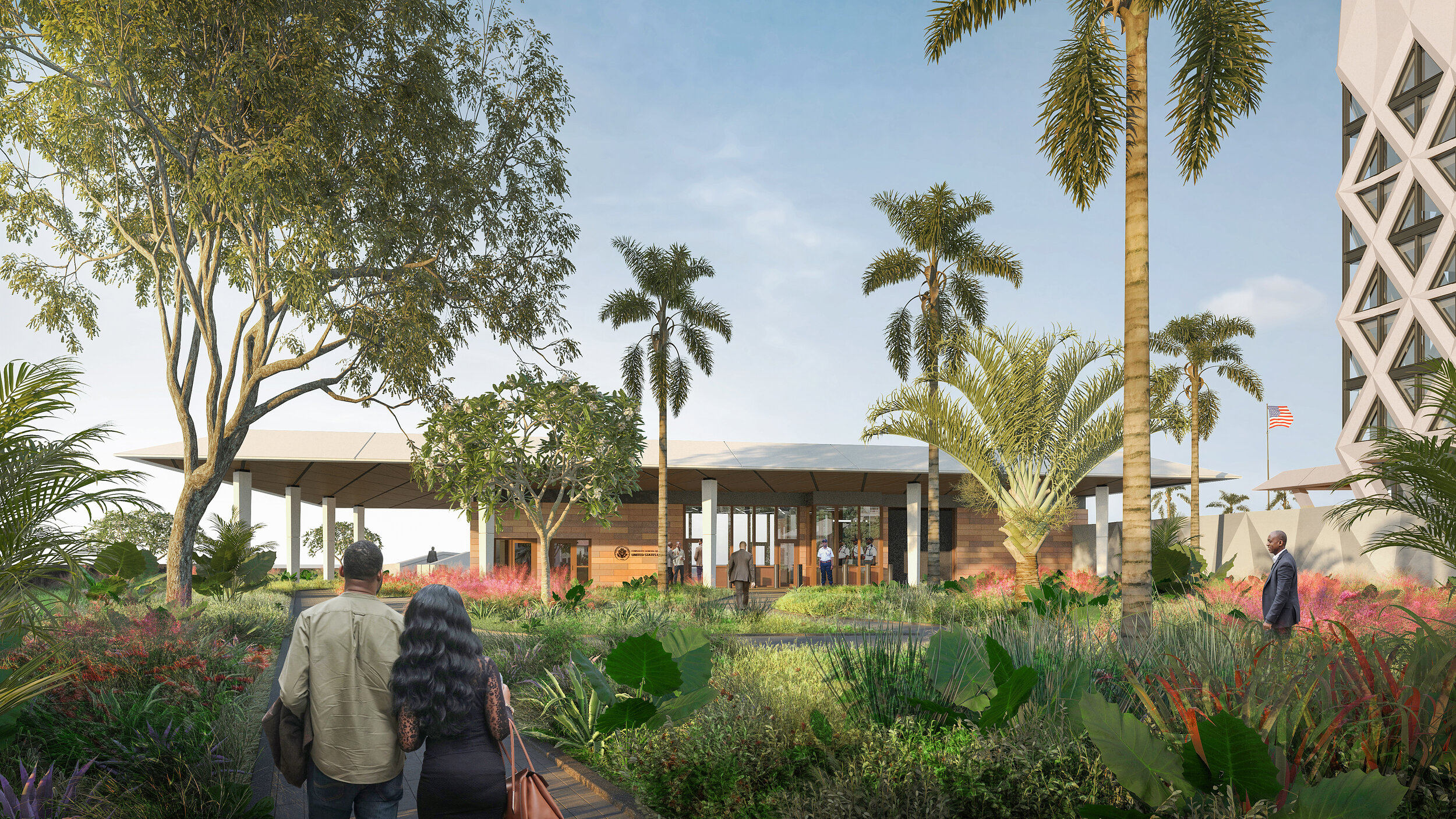A highly detailed 3D rendering showcases a modern single-story house nestled in a lush, tropical setting. The flat, white roof extends significantly outwards from the building's sides, supported by multiple square-shaped white pillars. The light brown walls, resembling natural wood, are accentuated by large glass panels set into brown wood frames. Leading up to the house, intricate walkways bordered by railings are flanked by a variety of tropical plants, including ferns and tall palm trees. Above, the sky is a light blue, noticeably brighter on the left side suggesting the sun's position. Towards the right, a tall white tower stands prominently. Parallel to the building, an American flag subtly waves in the background, identifiable by its blue square and red and white stripes.

In the foreground, a couple is walking towards the modern building. The man, dressed in a beige long-sleeve shirt, and the woman, carrying a brown purse and donning a black dress, appear to have dark brown skin, suggesting they might be African-American. The setting evokes the ambiance of a luxurious vacation resort, with its abundant trees, bushes, and colorful flowers with large leaves enhancing its beauty. The couple walks away from the viewer, heading towards the elegant structure with a glass entrance, adding a lively human element to the scene.